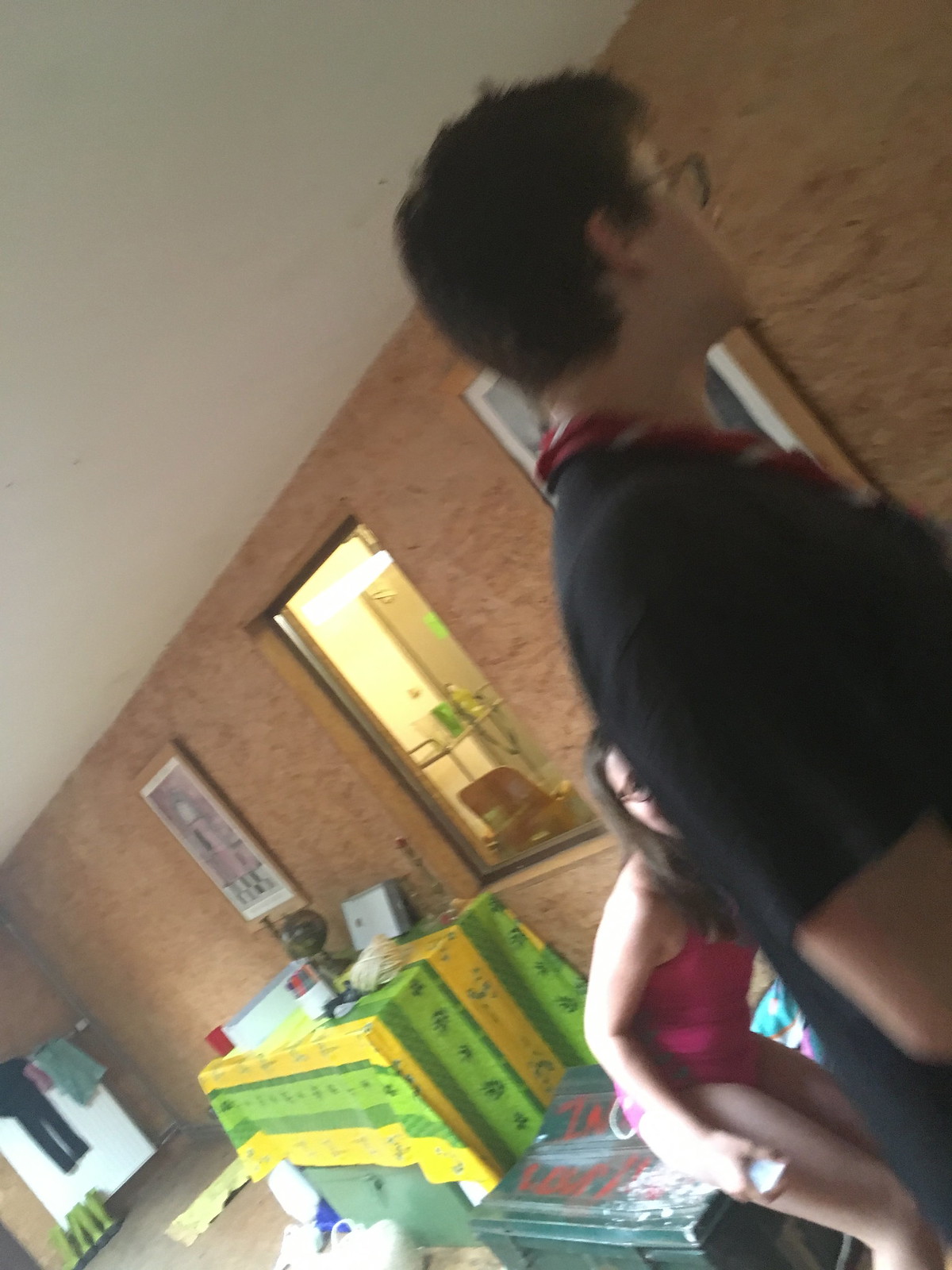The color photograph captures a candid moment inside a room with reddish-brown walls and a white ceiling, taken at a tilted angle. In the foreground to the right, a Caucasian man with short dark hair and glasses, wearing a black t-shirt, faces away from the camera, his face partially visible in profile. Behind him, a young woman with long brown hair and glasses, dressed in a bright pink sleeveless shirt and pink underwear, holds a phone in her right hand and appears to be smiling. She is leaning forward, seemingly about to sit on a large green plastic box with a lid adorned with red paint and writing. The background features a table draped with a green and yellow striped tablecloth, topped with various objects. Behind the table, a framed poster in pink, gray, and black hues is mounted on the wall. To the far left, rubber boots rest against the wall next to a railing with hanging clothes. A glass window beside the table offers a view into an adjacent lit room, where a metal trolley with a red plastic seat is visible near the window.